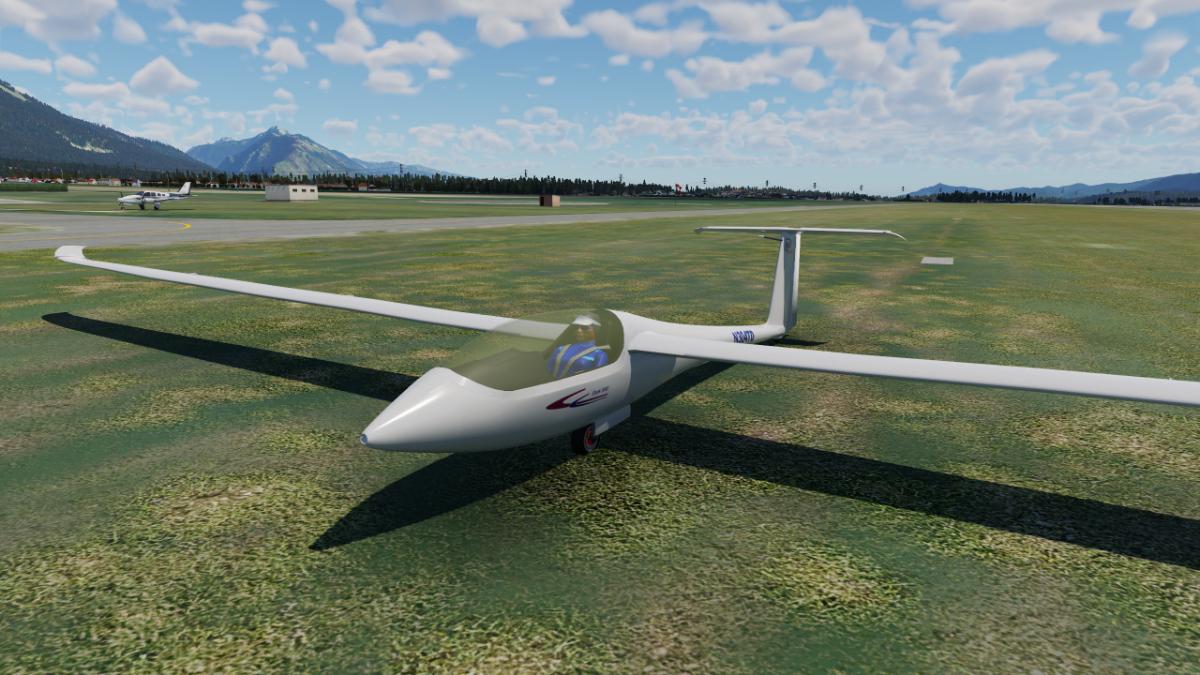In this detailed 3D-rendered image of an outdoor scene, we observe a futuristic-looking single-seat airplane, resting in a large grassy field in the foreground. The sleek, ultramodern design of the white plane is featured prominently, with its extremely long, thin wings—though part of the left wing is clipped off by the right edge of the frame. Inside the cockpit, there's a notably lifelike 3D model or possibly mannequin of a person dressed in a blue suit, suggesting it may not be piloted by a real individual. The scene captures a small regional airport setting with a long, paved runway extending from the upper left towards the middle right, surrounded by lush greenery. In the distance towards the left, another more conventional plane is visible, partially obscured by the grass. The background showcases expansive, low-lying mountains under a picturesque partly cloudy blue sky, adding a serene ambiance to the sunny day depicted in this meticulously crafted 3D model.